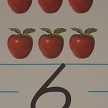This image features a neat arrangement of six bright red apples, organized in two rows of three against a white background. In the top row, the apples are partially visible, showing just the bottom halves, while the second row displays three whole apples. Each apple is adorned with two green leaves and boasts a shiny white spot indicating light reflection. Below the apples runs a solid light blue line, stretching horizontally across the image. Directly beneath this blue line sits a bold, black number '6,' slightly oversized compared to the apples, with its bottom portion cropped. The number '6' is flanked by short blue lines on either side, reminiscent of guidelines found in children's handwriting practice books.